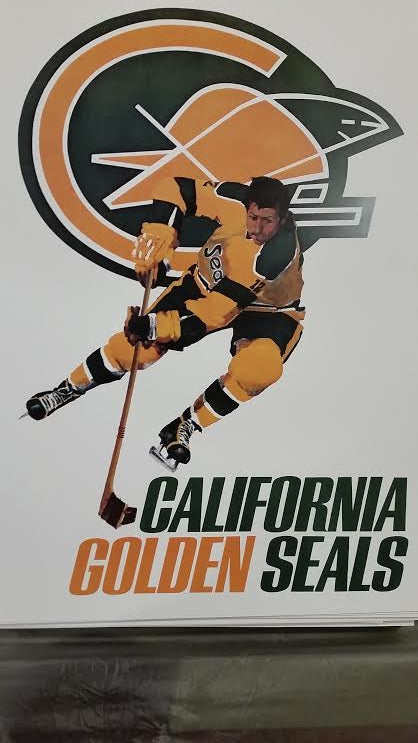The image is a poster or ad installed on a wall, featuring a professional hockey player prominently in the center. The bottom 10-20% of the image is a simple gray background, while the rest of it has a white background. At the top is a logo with a black background depicting a scene of the sea with abstract yellow, white, and black designs. Overlaying this logo, a hockey player is depicted in action. 

The player is dressed in a yellow jersey with black and green accents, green shoulder pads with white borders, and black shorts with a yellow or white stripe on the side. He wears black skates with black and yellow gloves and yellow knee pads. His serious, focused face suggests he is in his early 30s and has short black hair. The player is shown aggressively skating and leaning to the right, without a helmet, seemingly in control of the hockey puck that is at the end of his yellow and black-taped hockey stick.

At the bottom of the poster, the text reads "California Golden Seals," with "California" in black, "Golden" in a golden yellow color, and "Seals" in black or dark green.